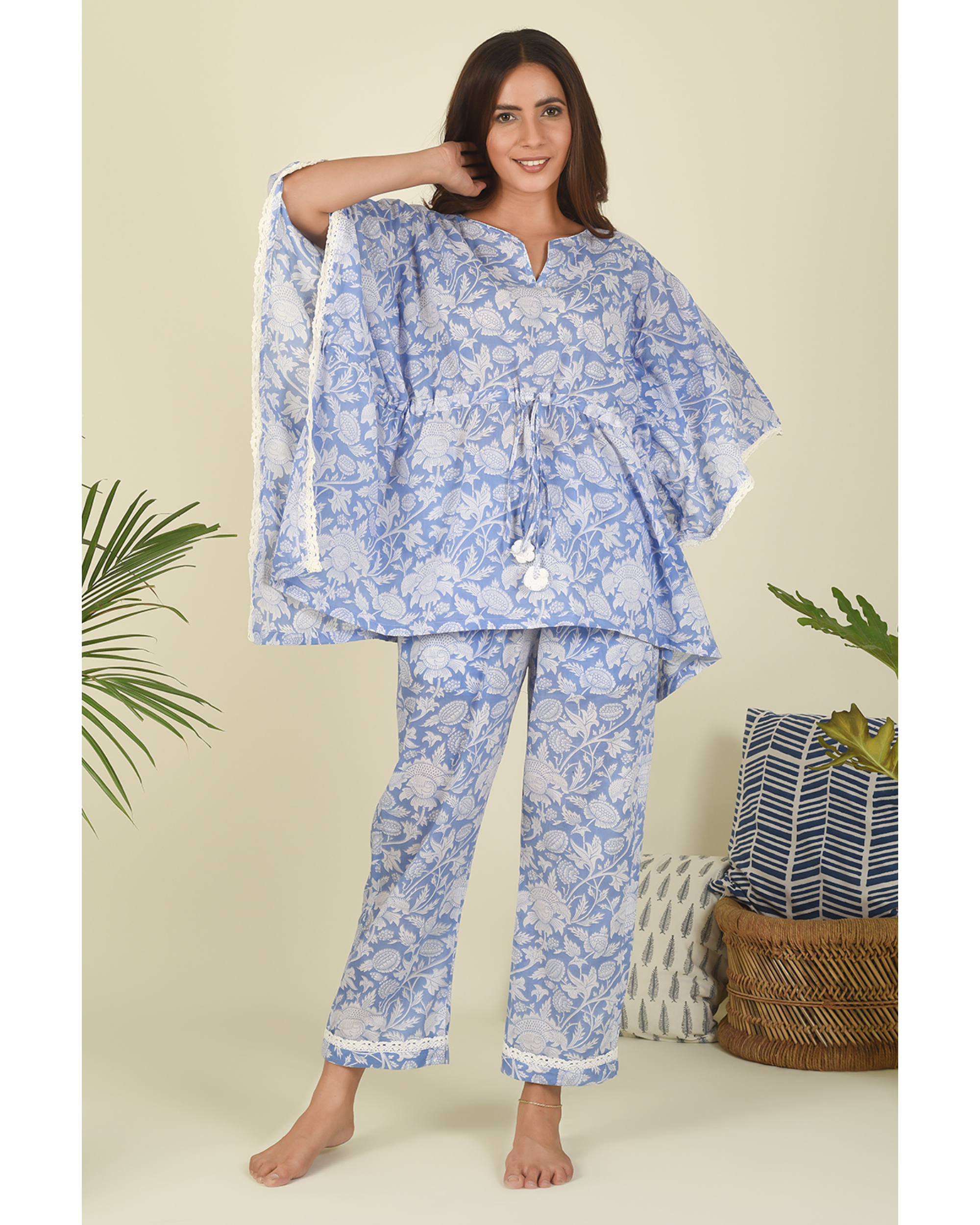A woman is posing and modeling an outfit in the center of the image. The background features a yellowish beige color that blends seamlessly from the floor to the wall. In the lower right-hand corner, there is a brown wicker basket with a blue and white striped pillow on top. Adjacent to the basket, to the left, is a white pillow adorned with a pattern of long gray leaves. 

The woman has long brown hair parted in the middle and she is smiling at the camera. Her right arm is bent at the elbow, with her hand resting behind her head as she holds her hair back. She is barefoot and wearing a flowing light blue shirt with white designs, which features very large, poncho-like sleeves and white tassels hanging down from it. She is also wearing matching pants that reach her ankles and have lace trim at the bottom. The ensemble gives the appearance of stylish pajamas. To the left and right of the woman, foliage, possibly from a fern or bush, adds a touch of greenery to the otherwise neutral setting.